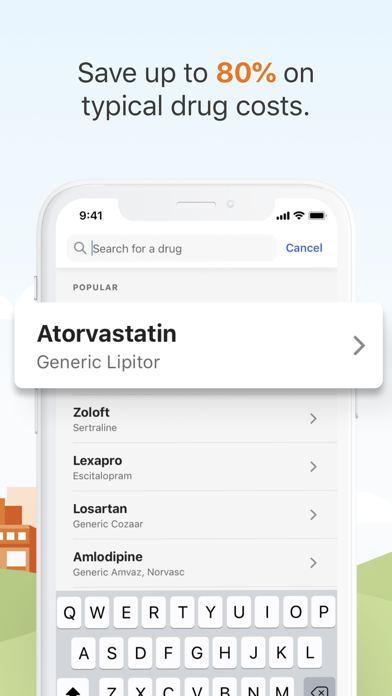In the image, an orange building with white-framed windows stands prominently against a backdrop of grassy green hills and a serene gray and blue sky. The scene captures a tranquil afternoon, with the lush landscape providing a vibrant contrast to the solid, warm tone of the building.